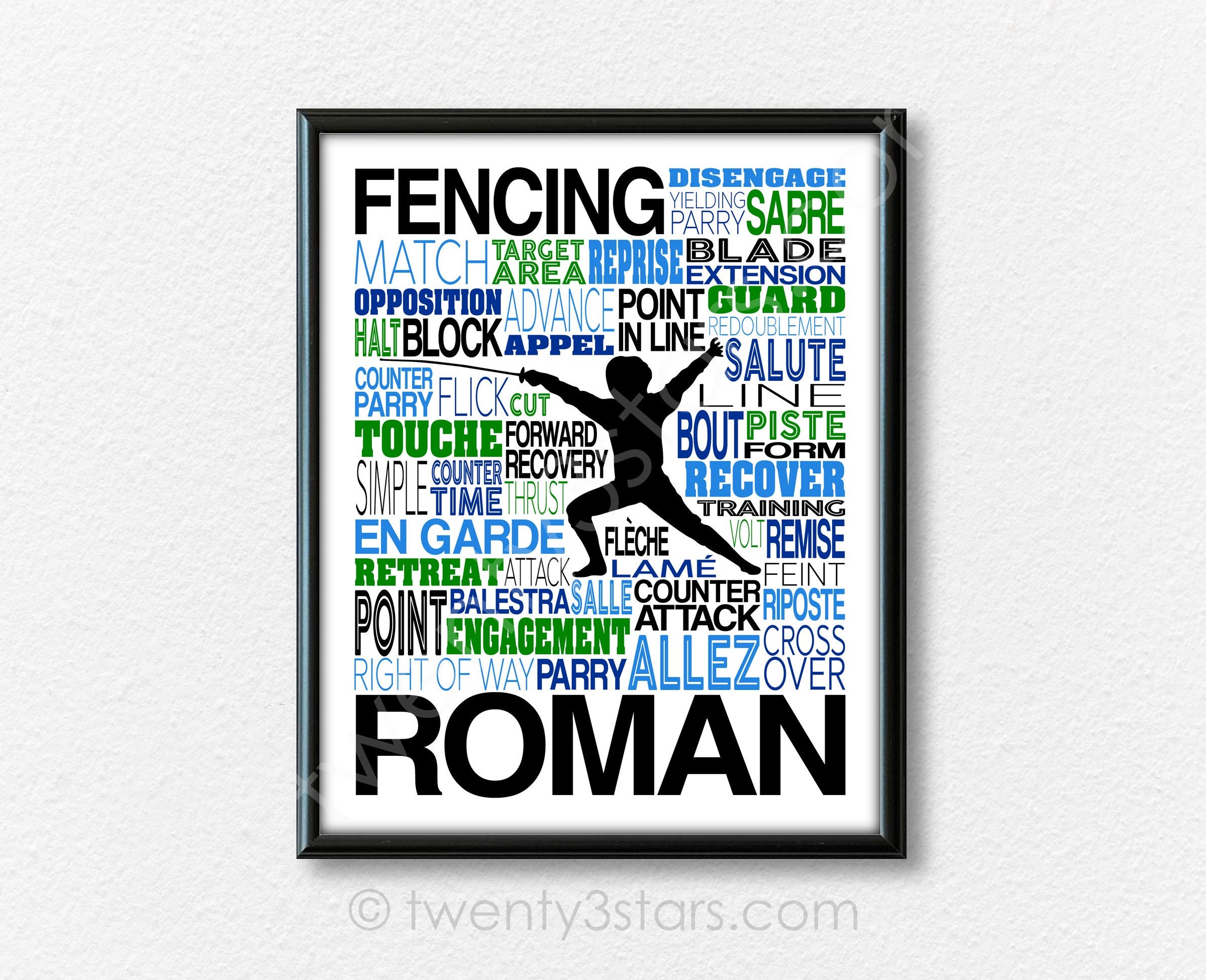The photograph shows a framed poster hanging on a white wall. The black plastic frame encases a white background featuring a black silhouette of a fencer in an athletic stance, with the right leg bent and the left leg extended. The fencer’s right arm, which holds a fencing sword, is extended forward. The poster prominently displays the word "Fencing" at the top, along with various fencing terms scattered around such as "disengage," "yielding," "parry," "saber," "blade extension," "match," "touche," "counterattack," "Roman," "cliche," "point and line," "right of way," "retreat," "attack," "engagement," "allay," "riposte," "guard," "recover," "bout," "opposition," "appell," "cut," "engagement," "piste," and "target area." These terms are written in different font sizes and colors, including green, blue, dark blue, and black text. At the bottom of the poster, in larger text, is the word "Roman." The entire composition gives a dynamic representation of the sport of fencing, highlighting essential terms and actions associated with it. Additionally, the lower portion discreetly mentions "23stars.com" alongside a copyright symbol.